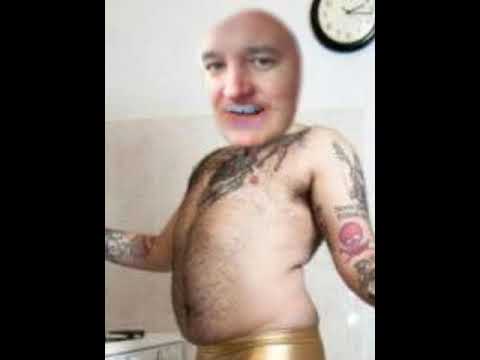This cartoonish image features a shirtless man, centered prominently, with detailed black and red tattoos on his arms, including a red skull. His head, appearing photoshopped and bald, is comically out of proportion and cut out against a white and tan wall. The unusual composition includes a clock in the upper right corner, showing the time as 2:15. Colors in the image range from white, black, off-white, tan, pink, purple, gray, to gold, with the setting possibly being a kitchen or living room. The man stands with open arms, clad only in underwear, adding to the surreal and slightly bizarre nature of the scene.